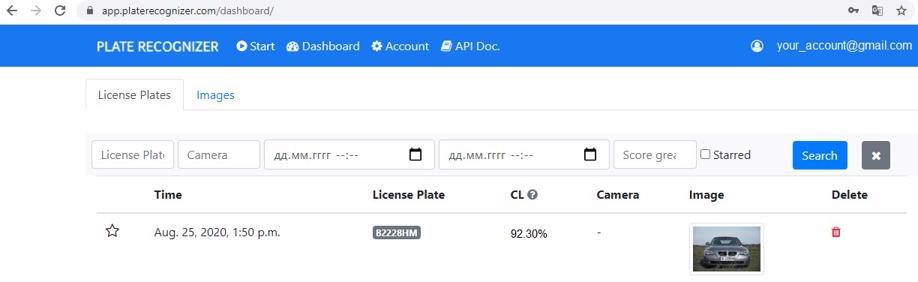The image is a screenshot of a computer screen displaying the dashboard of the website "appplaterecognizer.com." At the top of the page, beneath a gray address bar, a long blue navigation bar spans across the screen featuring the "Plate Recognizer" logo, accompanied by several icons. 

On the left of this blue bar, there's a circular icon with a right-facing triangle labeled "Start," next to the word "Dashboard." Further to the right is a bolt symbol, labeled "Account," followed by an icon resembling a sheet of paper or book, labeled "ApiDoc." 

On the far right side of the blue bar, there's an icon of a person inside a circle, next to the text "youraccount@gmail.com." 

Directly beneath the blue bar are two horizontal boxes. The first box is labeled "License Plates" and the second, longer box next to it is labeled "Images" in blue.

Below these boxes is another row containing multiple smaller boxes. The visible boxes are labeled "License Plate," "Camera," "Score," and "Start," among others that are unclear. Adjacent to these boxes on the right side is a blue "Search" button and a gray square with a white "X" inside it.

Further down, the page features another row containing columns with headers in dark black text. The columns are labeled "Time," "License Plate," "Camera," "Image," and "Delete." 

At the very bottom of the screen, there is an entry marked by a gray star on the bottom left corner. Next to it, the date is displayed as "August 25th, 2020, 1:50 p.m.," followed by a description: "Gray car facing the camera."